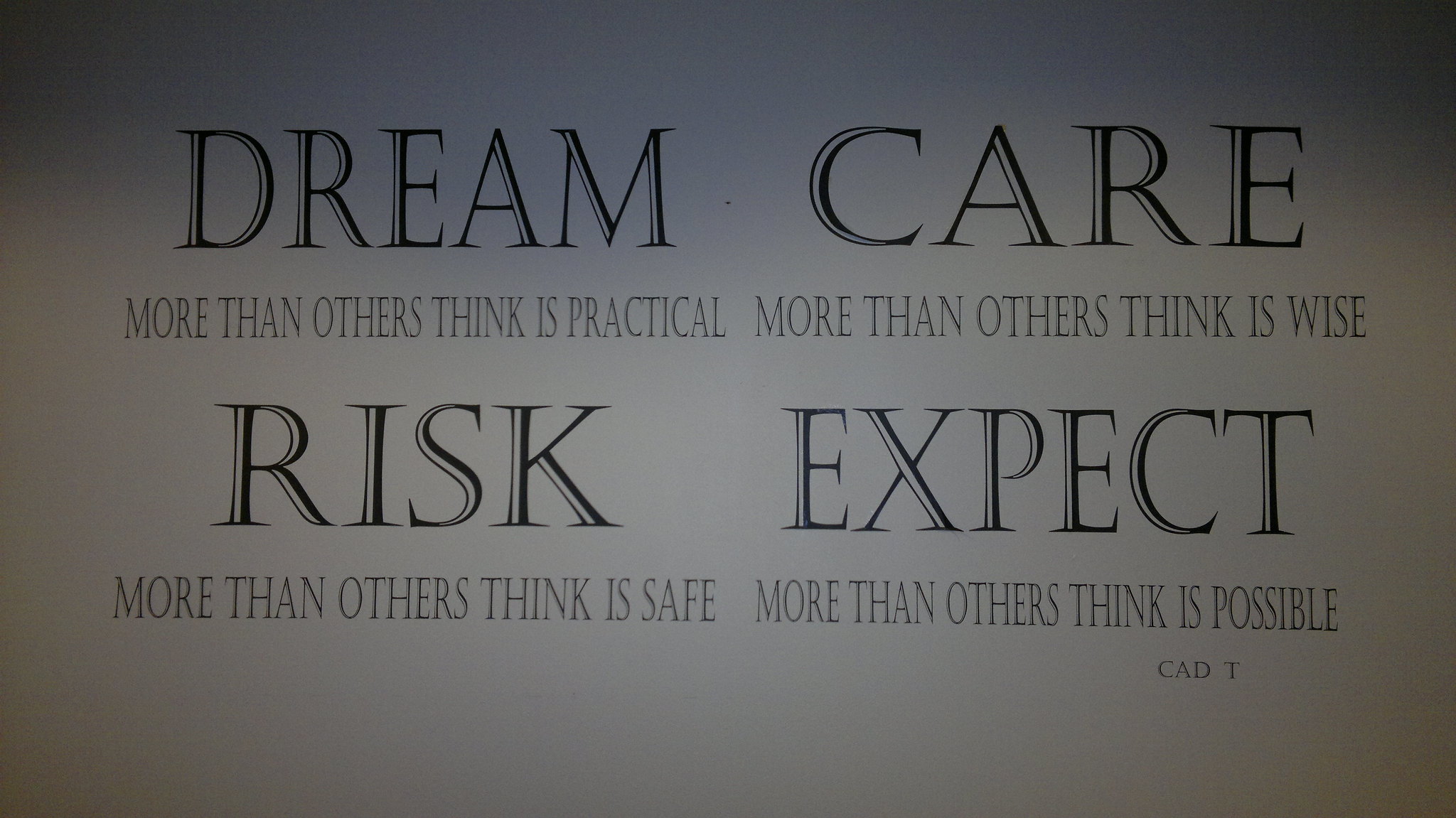The image features an inspirational quote on a simple white background with a subtle black shading at the top. Four key words—"DREAM," "CARE," "RISK," and "EXPECT"—are prominently displayed in large, bold, all-capital black letters. Each of these words is followed by a corresponding motivational phrase in smaller black letters: "more than others think is practical" under "DREAM," "more than others think is wise" under "CARE," "more than others think is safe" under "RISK," and "more than others think is possible" under "EXPECT." In the bottom right corner, the letters "CAD T" appear in small gray font. The overall message encourages readers to push beyond conventional limits in various aspects of life.